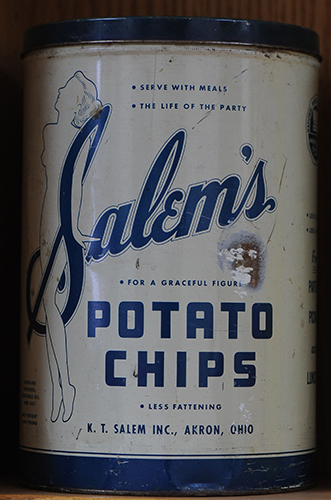This photograph showcases a nostalgic, vintage can of Salem's Potato Chips, reminiscent of the era when such treats were delivered directly to one's doorstep. The brand prominently displayed is "Salem's Potato Chips," with "Salem's" written in an elegant script font from which the outline of a woman emerges. She is delineated in blue, with her long hair styled in a bun. Her silhouette, appearing unclothed except possibly for a pair of undistinguishable shoes, adds a unique, artistic flair to the design.

The brand name "Salem's Potato Chips" is emblazoned in a rich dark blue color, matching the can's dark blue lid and base. The body of the can is a light gray, constructed from metal, giving it a sturdy, timeless appearance. Additionally, the inscription “Produced by KT, Salem, Inc., Akron, Ohio” indicates its place of manufacture, adding to the vintage charm and historical context of the piece.